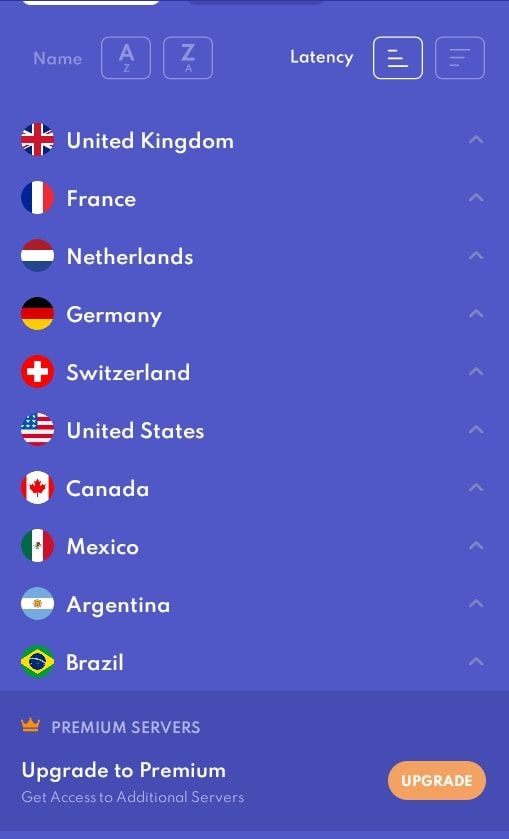**Detailed Caption:**

This image is a screenshot from an unidentified app, as the top portion including the app's name has been cut off. The app's interface features a purple background with the names of various countries listed and arranged in order of latency. The country names are displayed in a crisp white font and each name is accompanied by its national flag enclosed in a circle. The countries listed are: 

1. United Kingdom
2. France
3. Netherlands
4. Germany
5. Switzerland
6. United States
7. Canada
8. Mexico
9. Argentina
10. Brazil

Below this list, there is an option inviting users to upgrade to premium services, providing access to additional servers. Next to each country's name, there is a clickable tick bar, allowing users to explore further topics or subtopics related to the listed countries. At the top of the display, there are additional buttons, such as one for arranging the countries alphabetically from A to Z, though this option is not currently selected. The user is operating the basic, non-premium version of the app.